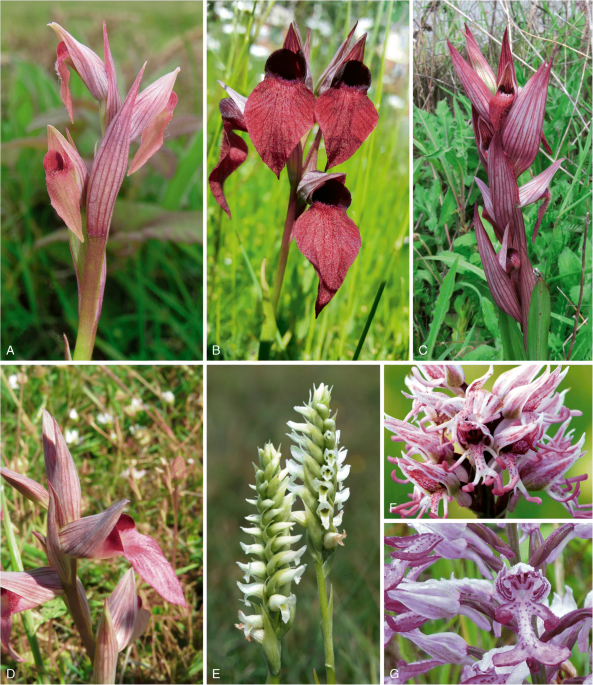The image is a detailed and vibrant vertical collage, divided into five vertical rectangles and two horizontal rectangles. The collage predominantly showcases various tropical plants and flowers, each vividly set against a backdrop of lush greenery. The top three vertical rectangles are segmented evenly, displaying different angles of spiky, pink, conical flowers with flat, broad leaves and pointy tips. These flowers, adorned with a red tinge, stand out strikingly against the green grass background behind them. Specifically, the upper left image (A) and the middle image (B) display similar pink flowers, but from distinct angles, while the top right image (C) features a darker, almost purplish variant of the same flower.

In the bottom portion, the left vertical rectangle (D) repeats the flower featured in (A), maintaining the theme of spiky pink petals. Adjacent to it is a horizontal rectangle (E) containing a white flower with green and pink hues, markedly different from the others in the collage. To the right, the bottom right corner of the collage is occupied by two horizontally stacked images (F and G). These smaller pictures present clusters of pale pink, trumpet-shaped flowers, their light color contrasting against the richer tones above.

Overall, the collage creatively captures the allure and variety of tropical flora through its meticulous arrangement and vibrant imagery.